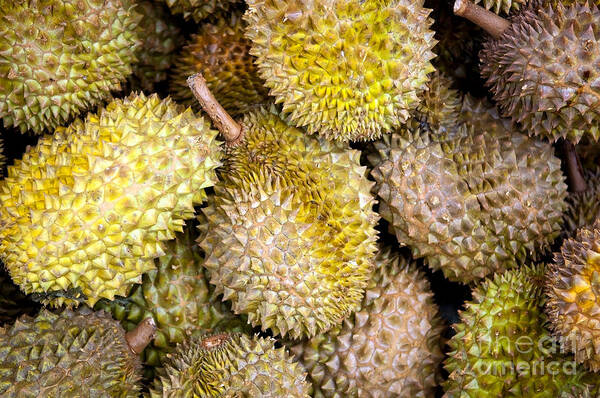The image features a plethora of spiky durian fruits, predominantly displayed in what appears to be a supermarket crate. The durians showcase a variety of colors, ranging from yellowish-green to various shades of brown, with some displaying a mix of these hues. Notably, a particularly bright yellow piece stands out on the left side near the center. The durian fruit at the center and at the top center of the image have a darker yellow color in the middle, with the surrounding areas shaded in light to dark brown. Several of the durians have their branches or twigs still attached; the center durian has its branch connected, while the durian at the top right has a brown twig attached. The bottom right durian is a striking blend of borderline yellow and lime green. Additionally, this corner of the image bears white, slightly transparent text, which reads "Fine Art America," suggesting it is part of a photograph from an art collection. The image captures the detailed texture of the durians' spiky shells, with their triangular, tooth-like points extending from each fruit, all amassed in a seemingly endless pile.